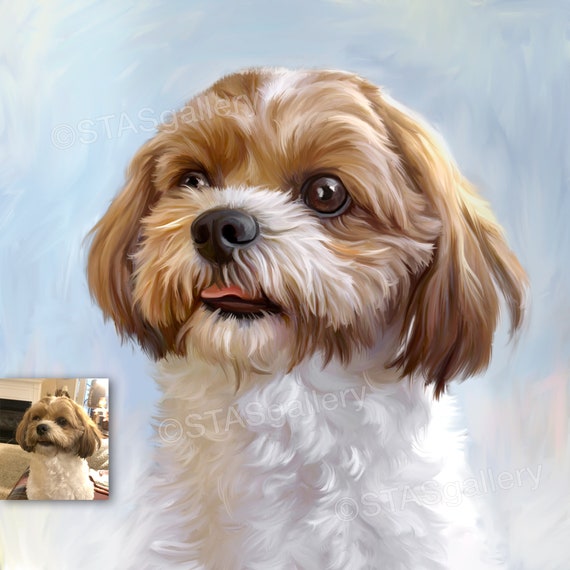This square image features an artistic print of a little Shih Tzu dog, closely capturing the pet's endearing facial details. The dog's face, with expressive large chocolate-brown eyes, is rendered with its mouth slightly open, showcasing its small tongue. The head displays a mix of light brown fur with a touch of white on the right side of its nose and under the chin, transitioning into its predominantly white upper body, though the legs are not visible. The background of the painting is an artistic blend of gray, blue, and white strokes, creating a visually soothing effect reminiscent of the sky. At the bottom left corner, there's an actual photograph of the same dog in a room setting, reinforcing the striking resemblance to the painted image. Additionally, a subtle diagonal watermark with a copyright symbol from "STAS Gallery" is visible in several spots across the image, adding an official touch to this well-crafted artwork.